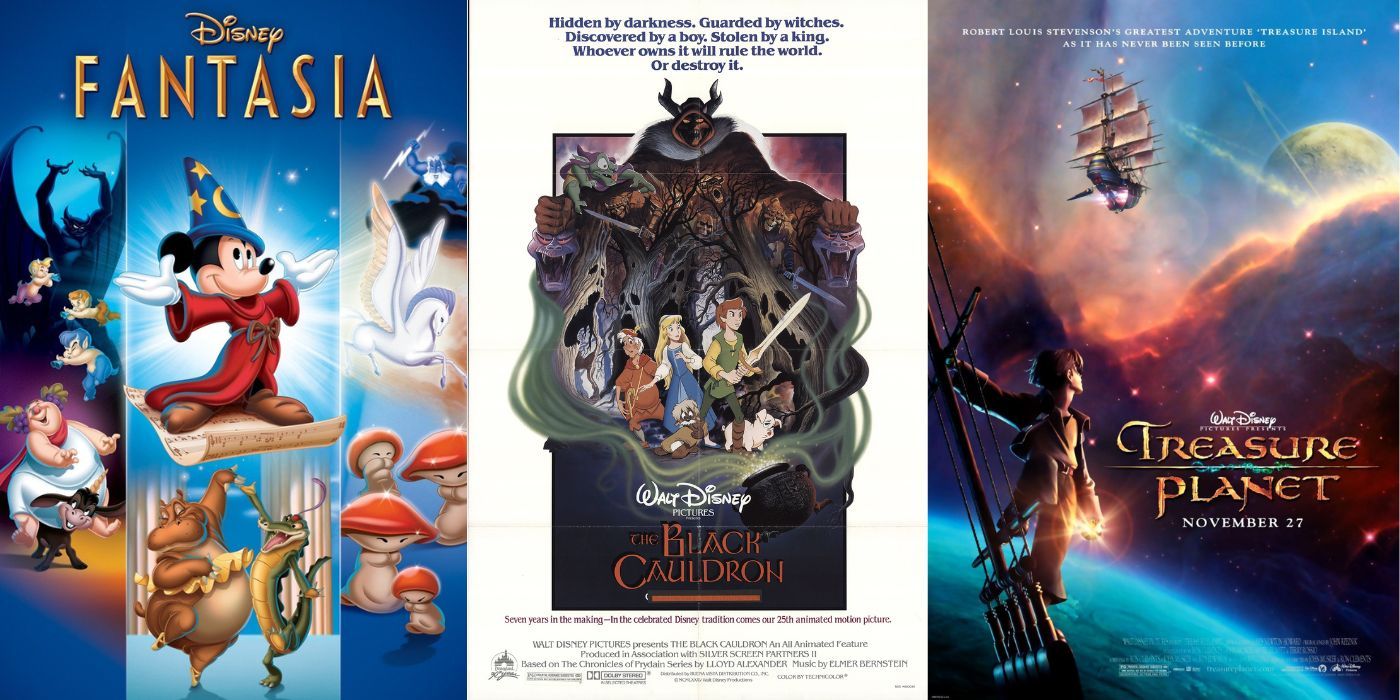The image features three Disney movie posters displayed side-by-side. On the far left, the poster for Disney's *Fantasia* is divided into three vertical sections. The top section showcases ethereal creatures like fauns and what seem to be flying entities. The middle section prominently features Mickey Mouse in his iconic wizard hat adorned with stars and a moon, clad in a red wizard robe, standing on a scroll of music with his arms outstretched. The bottom section illustrates a whimsical scene with a hippo in a tutu dancing ballet with a crocodile or alligator, alongside mythical characters such as a Pegasus, what appears to be Zeus wielding a thunderbolt, and charming little dancing mushrooms, all set against a predominantly blue background.

In the center, the poster for *The Black Cauldron* presents a dark, adventurous theme. It features a central figure identified as a young adventurer holding a sword, flanked by two animals, one of which is a pig. They appear to be navigating through a haunted forest with a menacing creature looming above them, arms spread wide. The poster includes an ominous tagline: "Hidden by darkness, guarded by witches, discovered by a boy, stolen by a king. Whoever owns it will rule the world or destroy it."

On the far right, the poster for *Treasure Planet* is set against a vivid scene of outer space with celestial elements. It depicts a young man hanging from the ropes of a pirate ship mast, gazing into the distance at another flying pirate ship. The backdrop displays a vibrant galaxy, a mysterious blue planet, and scattered space dust, lending a sense of adventure and exploration. The poster is dated "November 27th" and emphasizes the film's futuristic setting with elements of space and nautical themes intertwined.